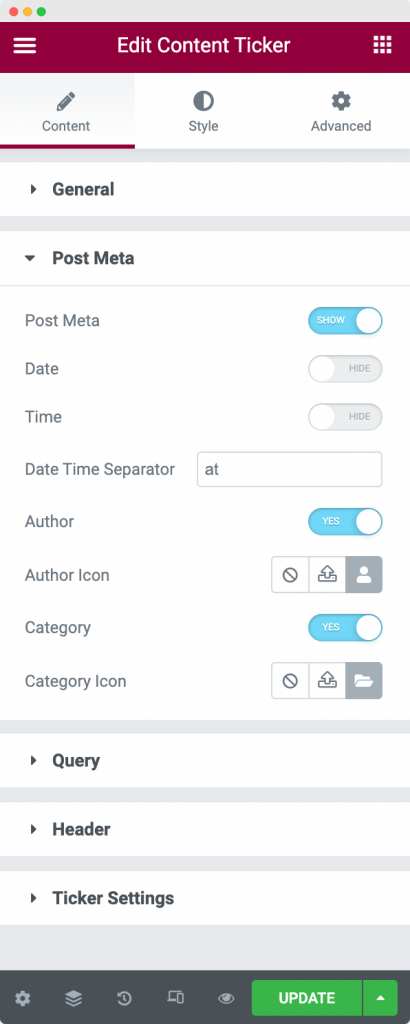A detailed screenshot from a smartphone displays a vibrant red background titled "Edit Concert Ticket." Immediately below the title are three icons displayed prominently. Next, the word "General" is shown in bold black letters. Further down, the text "Post Media Meta" is also highlighted in black. Below this, there is a "Post View" field accompanied by a toggle switch for user interaction. Continuing down the screen, a list of labels is visible: "Date," "Time," "Date," "Time," "Separator," "Author," "Author Icon," "Category," "Category Icon," "Query," "Header," and "Ticker Settings." Each function appears methodically listed, reflecting detailed customization options. The bottom of the screenshot is defined by a solid black border featuring a prominent green "Update" button, inviting the user to save any changes made.